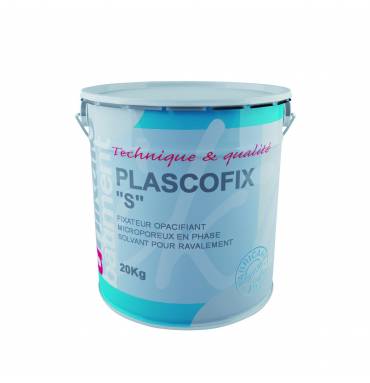This image features a detailed close-up of a smaller pail, likely associated with paint or a paint-related product. The pail has a blue, teal, and white color scheme with a white lid on top, and on the front, a white label partially obscures a cursive 'K'. The prominent text on the label includes "Technique and Qualité" in a reddish-pink font. Below this, in gray, it reads "Plascofix," followed by "S" in quotation marks. The French text underneath reads "Fixateur Opacifiant Microporeux Enphase Solvant Pour Ravalement." The pail weighs 20 kilograms, with "20 kg" displayed at the bottom left of the label. Additionally, there is a stamped teal or bluish-colored seal at the bottom right. The product seems to be related to paint, potentially a paint thinner or a fixative.